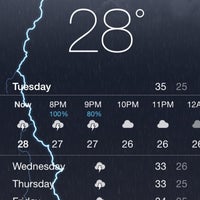Here is a detailed and cleaned-up caption for the given description:

---

The image showcases a weather application on a smartphone, likely an iPhone, though only the central section of the screen containing the weather information is visible. The display is detailed, with the current temperature prominently shown at the top in white text, indicating 28 degrees. Below that, it displays "Tuesday" with the highest and lowest temperatures being 35 and 25 degrees, respectively. 

The forecast section highlights the weather for the day with a timeline from 8 p.m. to 12 a.m. For 8 p.m., it shows a 100% chance of storms, represented by a cloud with a lightning bolt icon, and a temperature of 27 degrees. At 9 p.m., the probability decreases to 80%, with the same stormy icon and a temperature of 27 degrees. From 10 p.m. to 12 a.m., the icon changes to a cloud, signifying overcast conditions, with a temperature of 26 degrees.

Beneath this, the forecast for upcoming days is displayed, starting with Wednesday, continuing with icons of clouds and lightning bolts, and providing temperature ranges on the right side. The background of the app features animated rain falling from clouds, along with occasional lightning bolts, setting a dynamic and visually appealing interface.